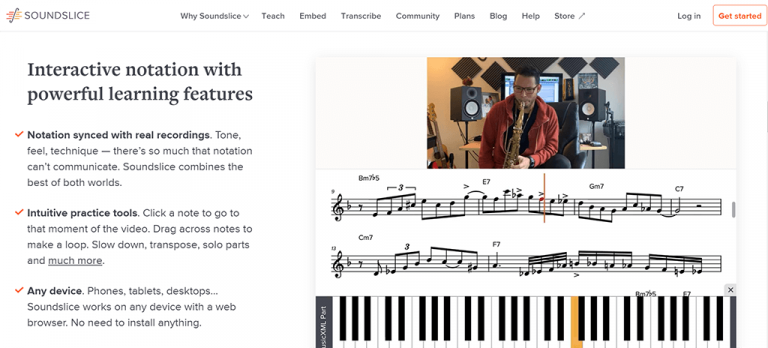The image showcases a webpage from the music website, Soundslice. The page has a clean, white backdrop with black text and various elements laid out methodically. In the top left corner, the Soundslice logo features prominently, consisting of the word "Soundslice" in uppercase black letters next to a stylized musical note intersected by red, orange, and yellow lines running horizontally.

At the top of the page, there is a navigational menu displaying several options: "Why Soundslice" (with a dropdown arrow), "Teach," "Embed," "Transcribe," "Community," "Plans," "Blog," "Help," and a "Store" marked with a pin. On the far right, there is a black "Login" button and an orange "Get Started" button within an orange-bordered box, indicating where new users can create an account.

The main content area is divided into two sections. The left side features textual information starting with a headline, "Interactive Notation with Powerful Learning Features," followed by three key bullet points: 

1. "Notation synced with real recordings" - Emphasizes the blend of timing, tone, feel, and technique that traditional notation alone can't capture.
2. "Intuitive, proactive tools" - Highlights features like clicking a note to jump to that moment in a video, looping sections, slowing down, transposing parts, and more, with interactive links for further exploration.
3. "Any device" - States Soundslice’s compatibility with phones, tablets, and desktops through any web browser without needing additional installations. 

To the right, an illustrative image is displayed. At the bottom of the image, there is a piano keyboard showing the keys for C, D, E, and F, with the F key highlighted in orange. Above the keyboard, music notation in the treble clef is seen, with the corresponding F note also highlighted in orange and underlined. At the top of the image, a photograph features a man playing the saxophone, flanked by two speakers.

The overall design of the webpage effectively combines functionality with a visually engaging representation of Soundslice’s capabilities, targeting musicians and educators seeking interactive digital tools.